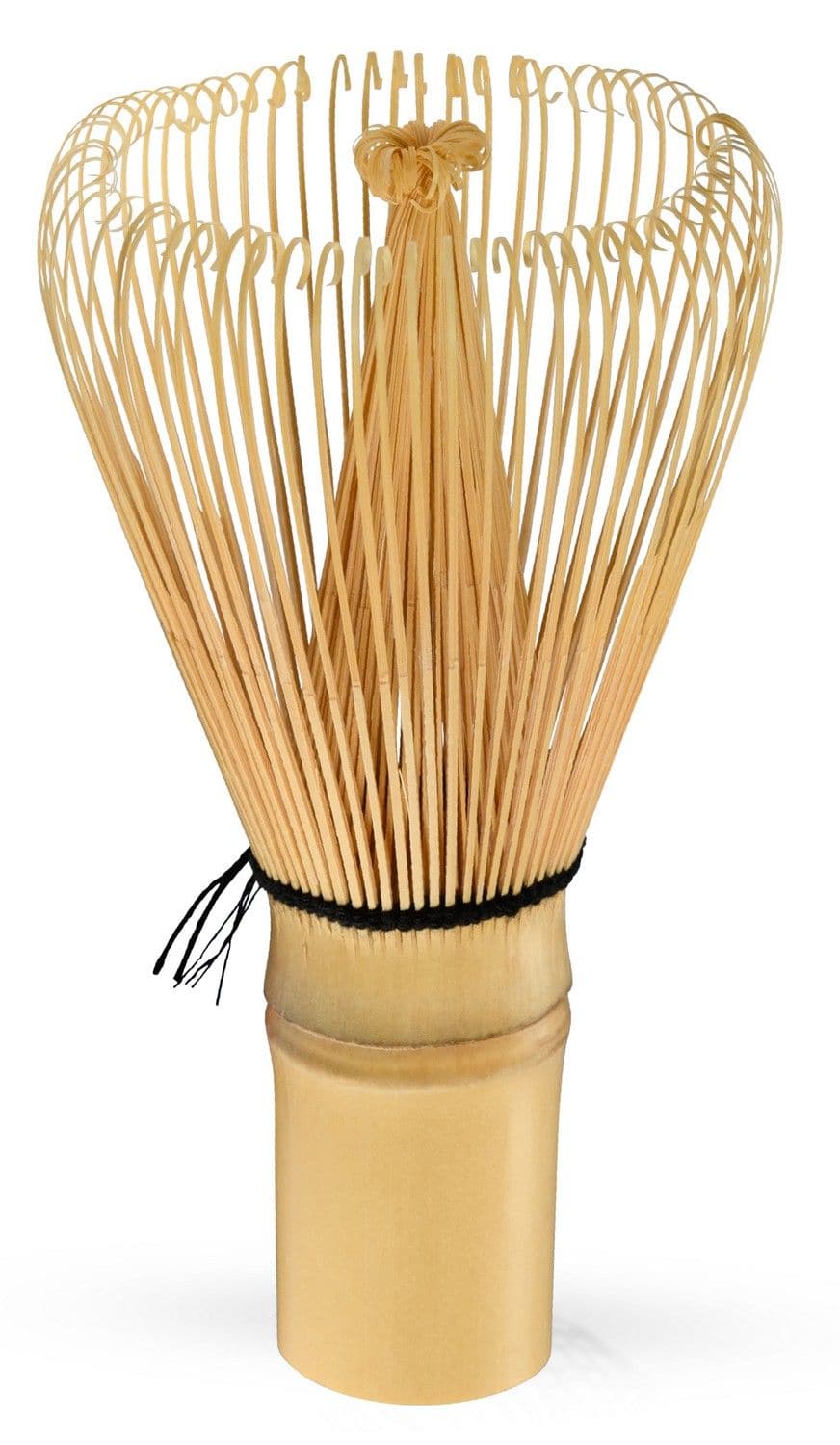This image showcases a delicate and intricate piece that appears to be a tool or an art object, centered in portrait mode with no background. The base of the item is a golden tube, possibly made of wood or plastic, adorned with a black threaded ribbon where it attaches to the handle. The handle itself is short and emerges from this tube, potentially made from a cream-colored material, either wood or plastic.

Above the handle, intricate craftsmanship is evident, resembling both a conical whisk formation and a blooming flower. Thin slivers of bamboo or wood, carefully sliced and curled at the ends, extend outward and inward from the center, creating a layered pyramid or tent-like structure. The inner strips form a conical shape in the middle, while the outer strands curl gracefully toward the top. This convergence of strands is held together at the base by black thread, adding to the aesthetic and structural integrity of the piece.

The artistry or purpose of this object remains ambiguous, but it features an elegant fusion of organic materials and thoughtful design, potentially serving as a brush, a decorative piece, or a unique tool.